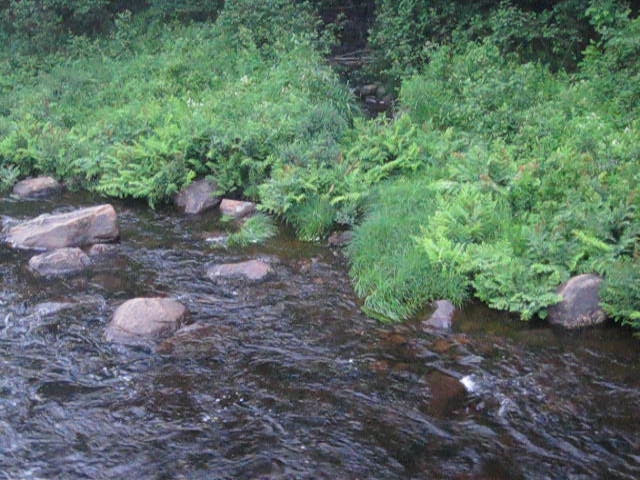The image depicts a shallow stream with dark gray to brown water, filled with visible ripples and bubbles. Numerous rocks protrude both above and slightly below the water's surface, some of which show partial submersion by the stream. The bottom half of the scene prominently displays these well-worn rocks, which exhibit various shades of gray, speckled with hints of blue and white. At the water's edge, vegetation appears to have grown up to and around the rocks, with ferns or similar plants extending into the stream. This vegetation ranges from light to medium green in the lower parts of the image and transitions to darker green foliage towards the background. There are patches of taller green grasses and shrubs, especially in the upper half of the scene, giving way to a more densely packed, darker background. Amidst the dark green foliage in the distance, there is a hint of a possible structure, with the faint outline of a roof barely visible through the trees. This overall daytime shot captures the tranquil yet subtly dynamic nature of the stream and its surrounding verdant environment.